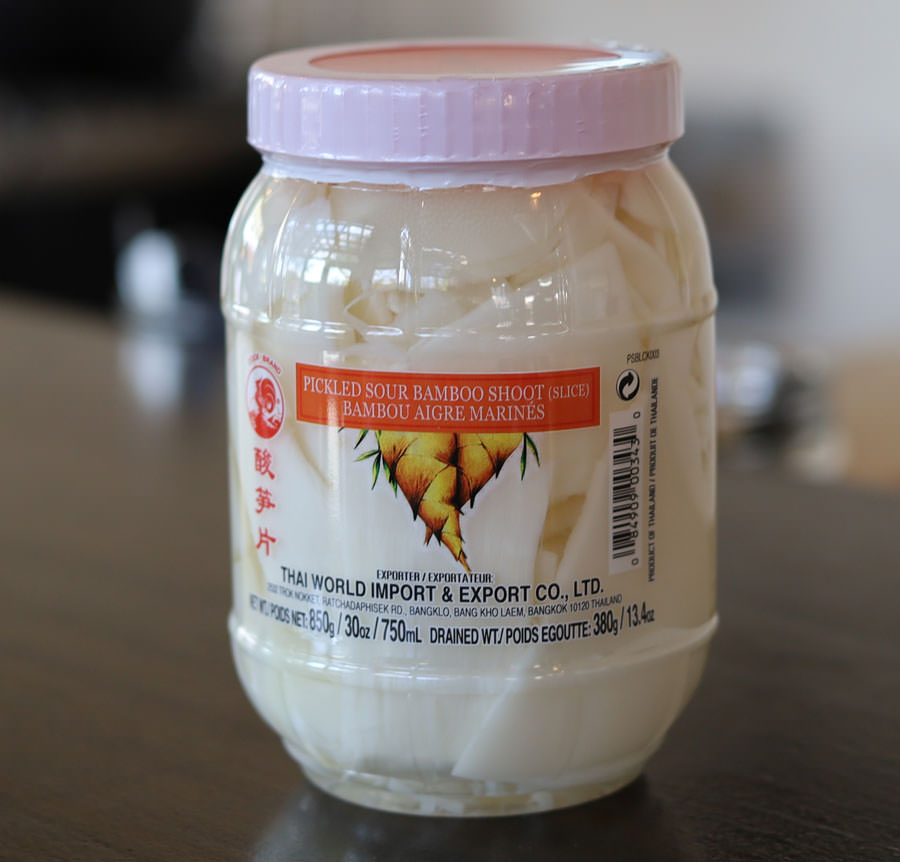The photo captures a white plastic jar, reminiscent of a mayonnaise jar, with a screw-off lid sealed by an intact safety wrapping and additional safety plastic. The jar sits on a dark wooden table, while the background is blurred, enhancing focus on the product. The jar prominently displays an orange label with white text that reads "Pickled Sour Bamboo Shoot (Slice)." Beneath this, the label includes additional information in a foreign language, and an illustration, rather than a photograph, depicting bamboo shoots, which slightly resemble large, triangular-shaped carrots with a curving shape. Additionally, the label notes "Thai World Import and Export Company LTD," and provides weight measurements: 850 grams, 30 ounces, and 750 milliliters. The right side of the label features a vertically oriented barcode and recycling symbol. Vertical text in what appears to be Chinese or a similar East Asian script is printed in orange alongside another small orange illustration. The photo is taken from a direct side view, emphasizing the detailed label against the indistinct backdrop.